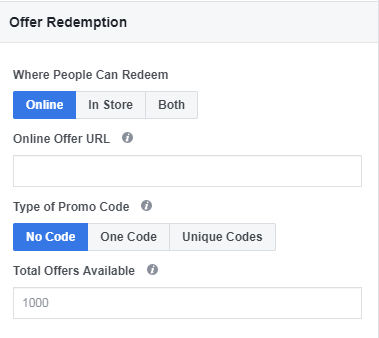The image displays a website section titled "Offer Redemption" prominently at the top. Beneath this title, the text "where people can redeem" is written in black. The layout includes a long rectangular area divided into three equally-sized boxes, labeled "Online," "In-Store," and "Both," in sequence. 

Adjacent to these, the section "Online Offer URL" is visible, accompanied by a gray circular icon with a lowercase "i" in the center, which provides additional information when clicked. Below this, there is a clear, rectangular input field.

Further down, the section labeled "Type of Promo Code" can be seen, also featuring the gray icon with the lowercase "i" for additional details. This section includes another set of three boxes, which are larger than the previous trio. The first box displays "No Code" in white text on a blue background. The second box is gray with darker gray text reading "One Code." The third box is a lighter gray with the phrase "Unique Codes" in a slightly darker gray font.

Finally, under the "Total Offers Available" heading—again marked with the information icon—a rectangular input box spans the width of the section, showing the number "1,000".